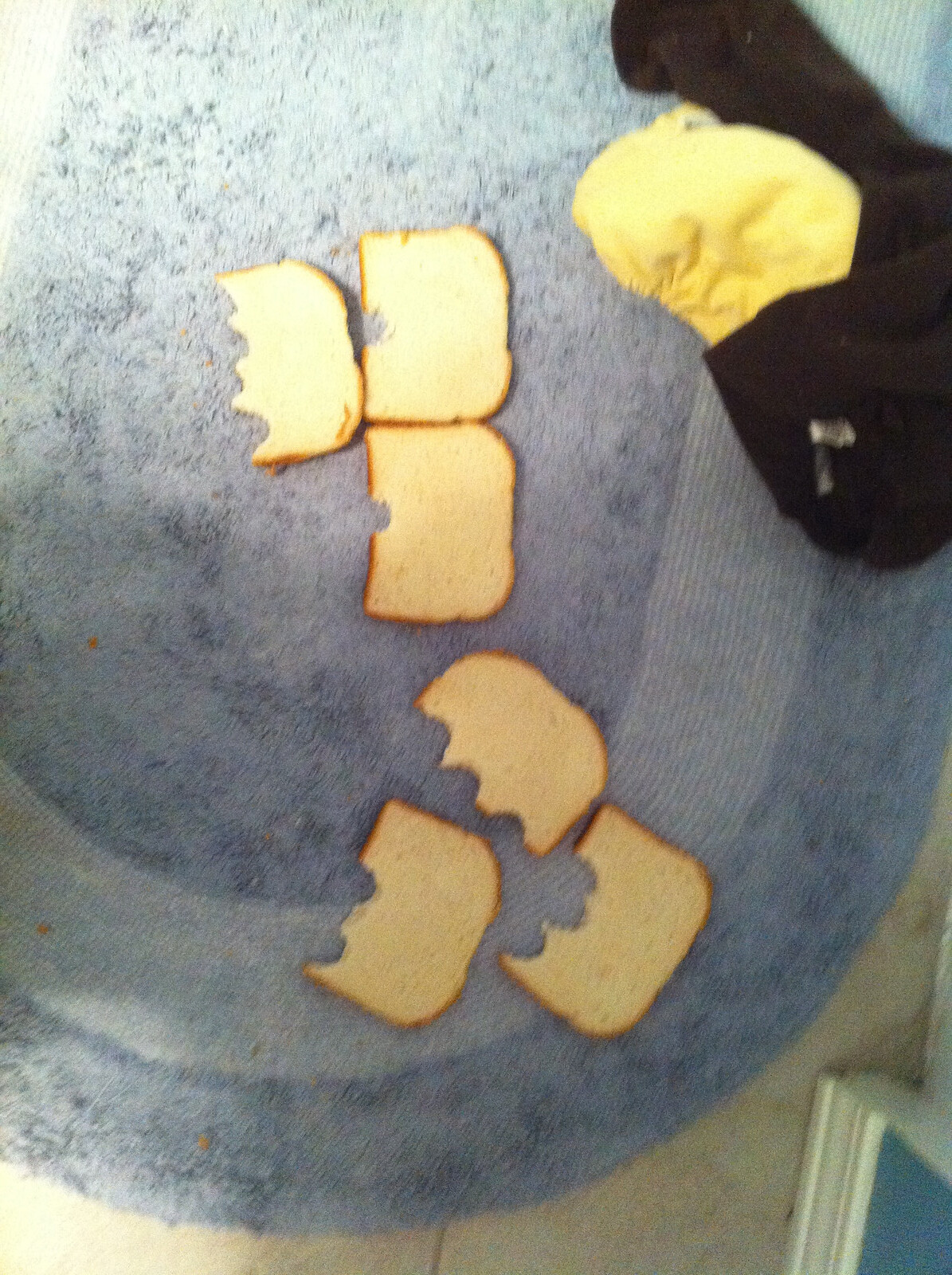The image depicts six slices of white bread, all of which have been partially nibbled, sitting on an oval blue bathroom rug. Four pieces have several bites taken out of them, while two have only one bite each. The rug appears slightly dirty and is situated on a light grey or beige tiled floor. In the top right corner of the image, a crumpled black and yellow piece of cloth or clothing can be seen. Additionally, the lower right corner shows part of a deep blue wall with white molding. The scene gives an impression of disorder, as if a child has taken bites out of the bread and then abandoned them on the rug.